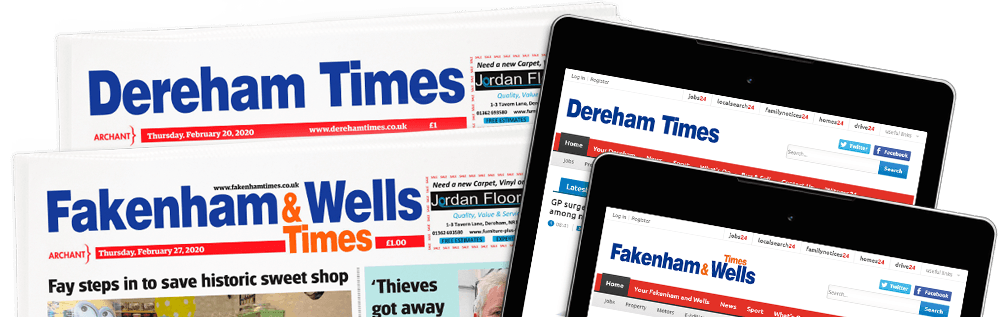This image showcases a close-up of several newspapers and their digital versions displayed on a tablet or a smartphone. The newspapers, titled "Derraham Times" and "Frankenham and Wells Times," are prominently featured. Headlines such as "Fay Steps Into Historic Sweetshop" and "Thieves Got Away" are visible at the top. Additionally, web interface elements from their respective websites are shown, including icons for Facebook and Twitter, a search bar, and a date stamp reading "February 20, 2020." One paper features a coupon for "Jordan Floor." The digital platforms mirror the layout of the physical newspapers, integrating modern connectivity with traditional news media.